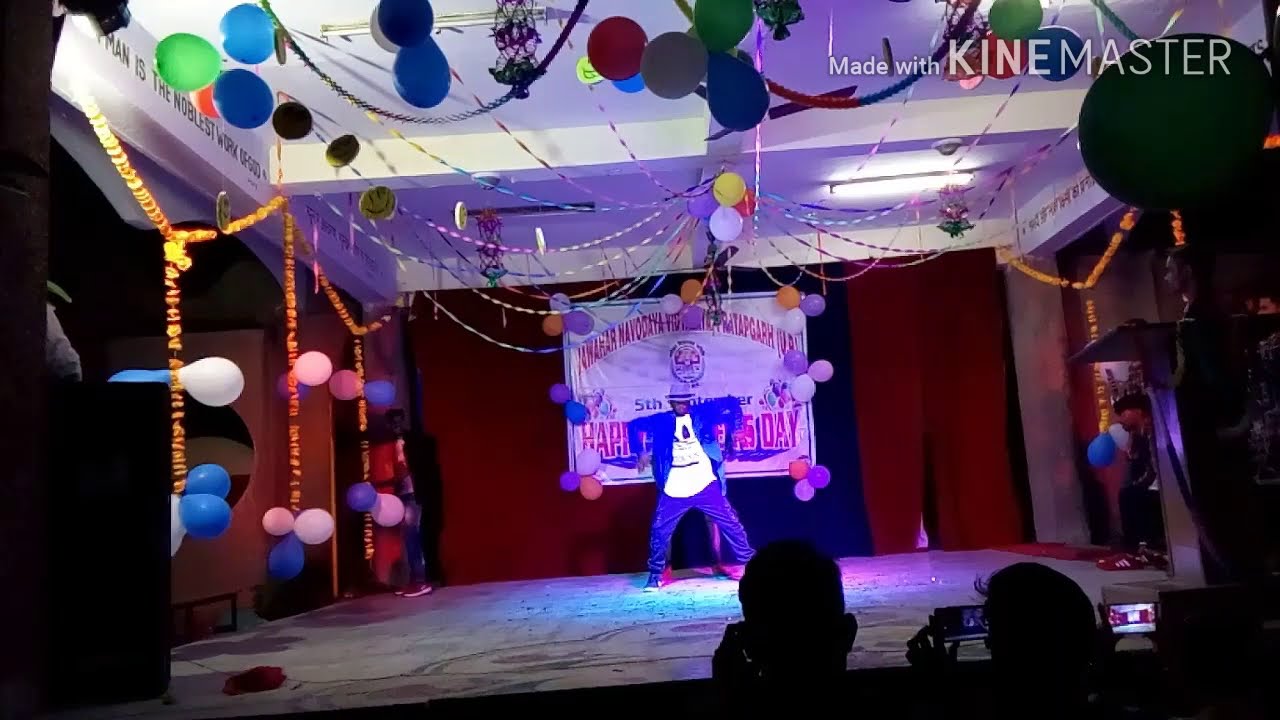The image showcases a lively celebration on a dimly lit stage with a purple hue. At the center, a Black man wearing a blue jacket over a white t-shirt, baggy dark blue pants, and blue sneakers or runners is enthusiastically performing. He sports a grey hat and his arms are bent at 90 degrees, appearing to be in mid-dance with his legs spread shoulder-width apart. Behind him hangs a large white banner with red lettering, though the exact message is unclear. The stage itself has scattered white cloth and surrounding decorations include streamers in various colors—purple, orange—and multiple balloons dangling from the bluish-white ceiling, which features fluorescent fixtures. On the left side of the stage, partially visible black lettering on a beam reads, "Man is the noblest work," though the rest is obscured. The background is adorned with blue and red curtains. The image also captures the heads of spectators and their devices recording the event, and another man stands to the right, attentively watching the performance. In the upper right corner, white text reading "Made with Kine Master" is printed on the photograph.